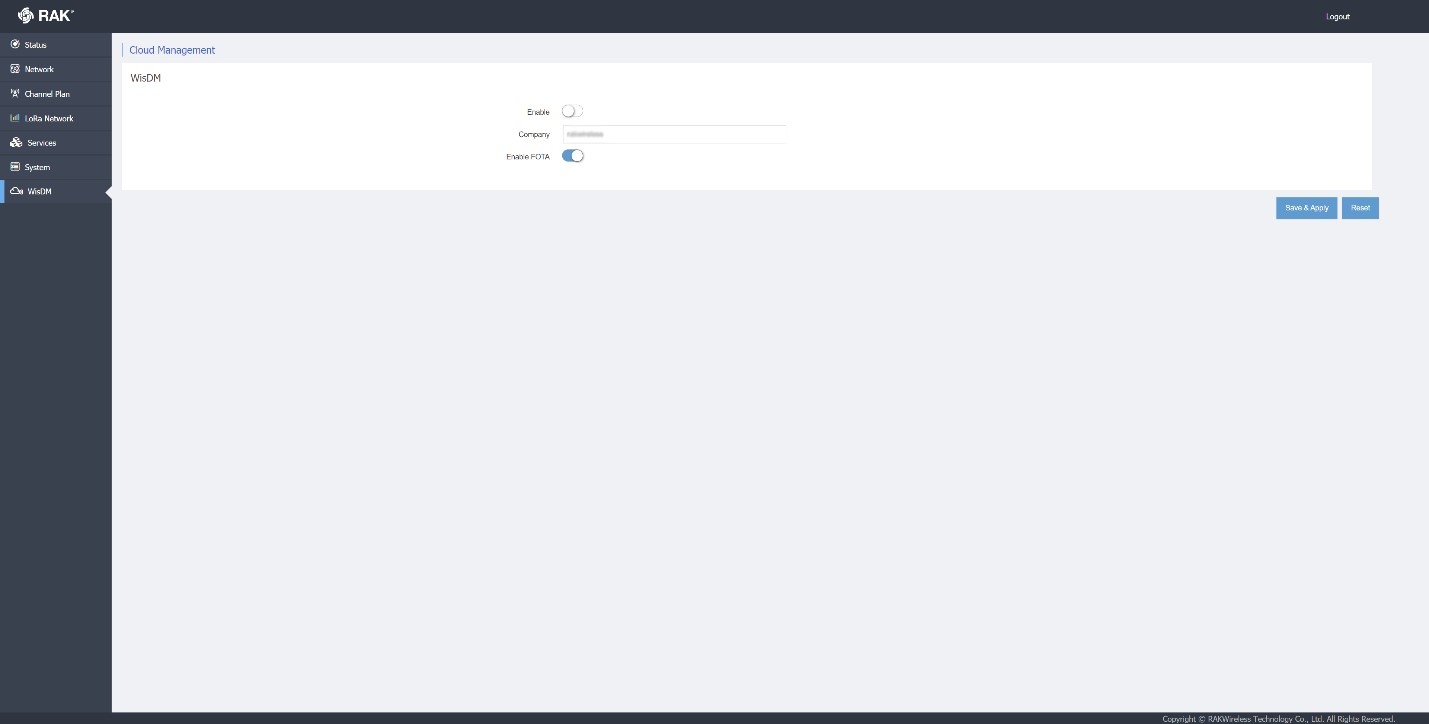The image displays a computer screen with a minimalist design. At the top, there is a very thin black banner, accompanied by a gray strip above it. Positioned to the left of the black banner is a logo featuring the capital letters "R-A-K," presumably representing the business name. On the far right of this banner, there appears to be either a login or logout button, depending on the user's status.

Along the left side of the screen, a vertical gray sidebar presents several navigation options: the first labeled "Home," followed by "Network." The third option is indistinct due to its small size. The fourth option is partially visible and seems to include the word "Network Service." The last option in this sidebar is highlighted with a blue line, indicating it is actively selected, and reads "Cloud Management." Beneath this selection, a small black symbol is present but difficult to discern.

In the main section of the screen, three fillable windows are displayed. Beside these windows are interactive elements, including a toggle button that is currently active. Below this are two small blue buttons, which are notably difficult to read due to their size. Overall, the design elements, especially the text and symbols, appear small and could be challenging for some users to view clearly.